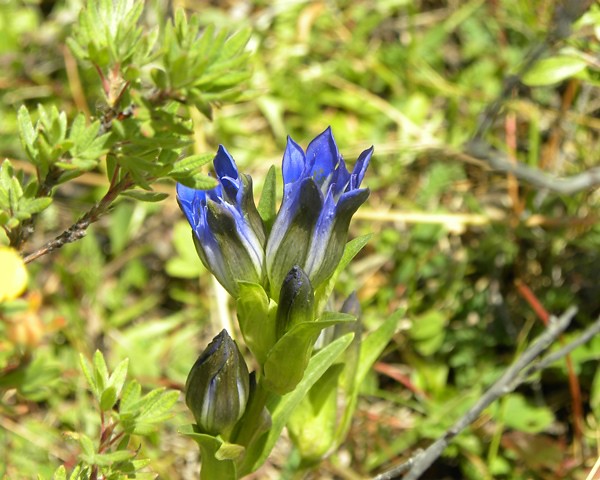In this early spring scene, a close-up captures the blooming stages of a purple-blue flower, similar to a camas flower. The main focus is on the central flower, which is just beginning to open, revealing its diamond-shaped petals. Surrounding it are four buds: the top two are starting to show their bluish-purple hue, while the bottom two remain tightly closed, encased in leaves. The flower and buds are set against a blurred, hazy green background typical of a forest or wooded area, with faintly discernible thin branches and small green leaves. The bright midday sun illuminates the scene, enhancing the vibrant springtime atmosphere where the flora is awakening.